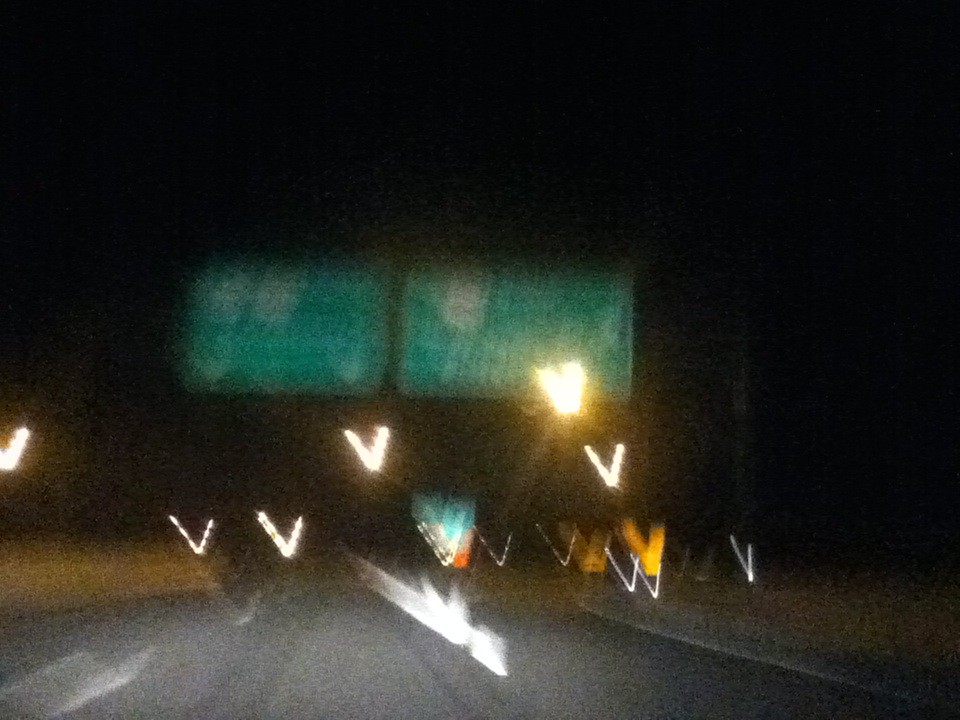This photograph captures a very blurry scene of a nighttime drive down a highway. The image, likely taken quickly from the passenger seat of a moving vehicle, features a pitch-black sky with no visible stars or moon. Central to the composition are two large, green overhead highway signs with shield-shaped markers, typical for indicating highway numbers and exits, though the writing is too blurred to read. Multiple sources of light – possibly streetlights and reflective signs – create bright, yellowish streaks and V-shapes across the photo, suggesting motion. These streaks further obscure any fine details, leaving only the impression of a dark, concrete road bordered by what appears to be grass or possibly dried vegetation on either side.